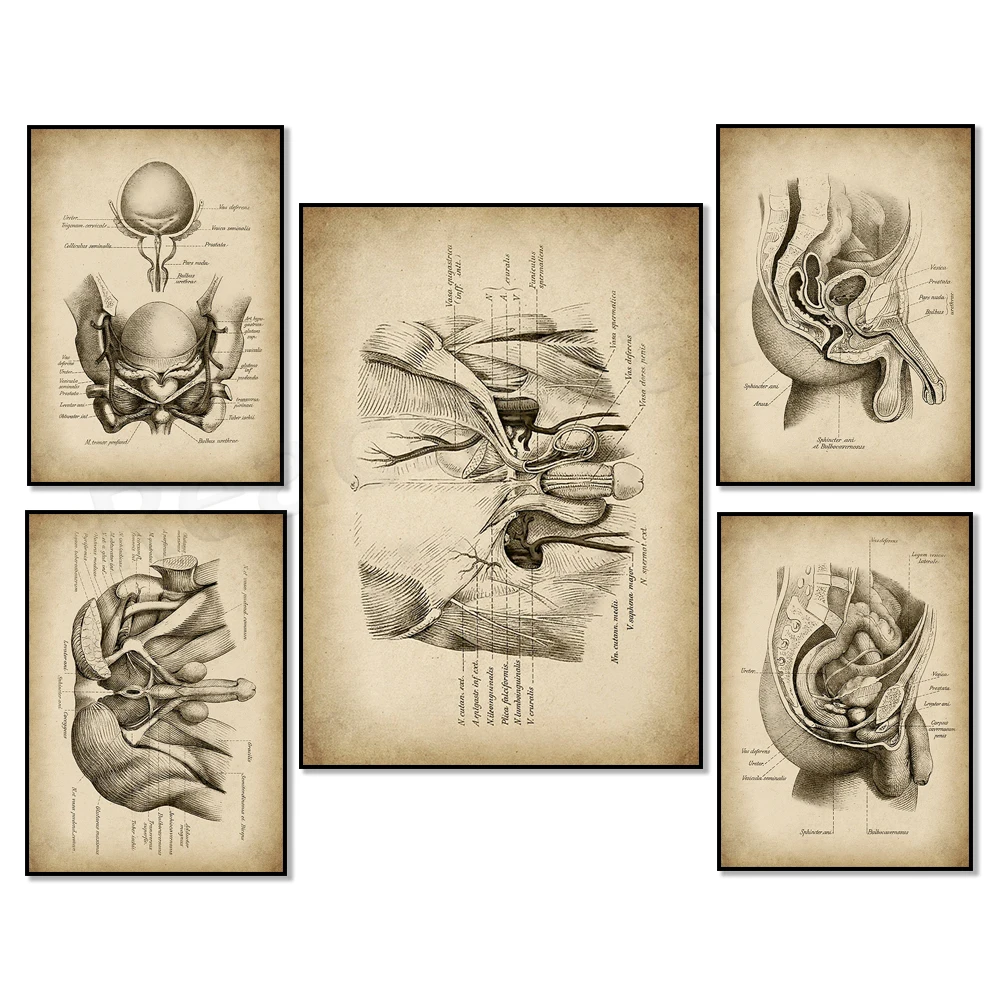The image depicts a detailed medical illustration featuring five distinct diagrams of the male reproductive and pelvic anatomy. Arranged with two images on the left, one prominent central image, and two on the right, the illustrations collectively showcase various views and cross-sections of male sexual organs, including the penis, testicles, scrotum, and surrounding pelvic structures. Each diagram highlights different anatomical features with precise labeling, although the text is too small and distant to read. The drawings, rendered in a tannish hue, emphasize both the internal and external perspectives, illustrating muscle, bone, and other tissues in a style typical of medical textbooks. The upper right image, for instance, focuses on the internal pelvic anatomy devoid of skin, while other images include detailed cross-sections that reveal the layers of muscle and bone within the penis and pelvic region.